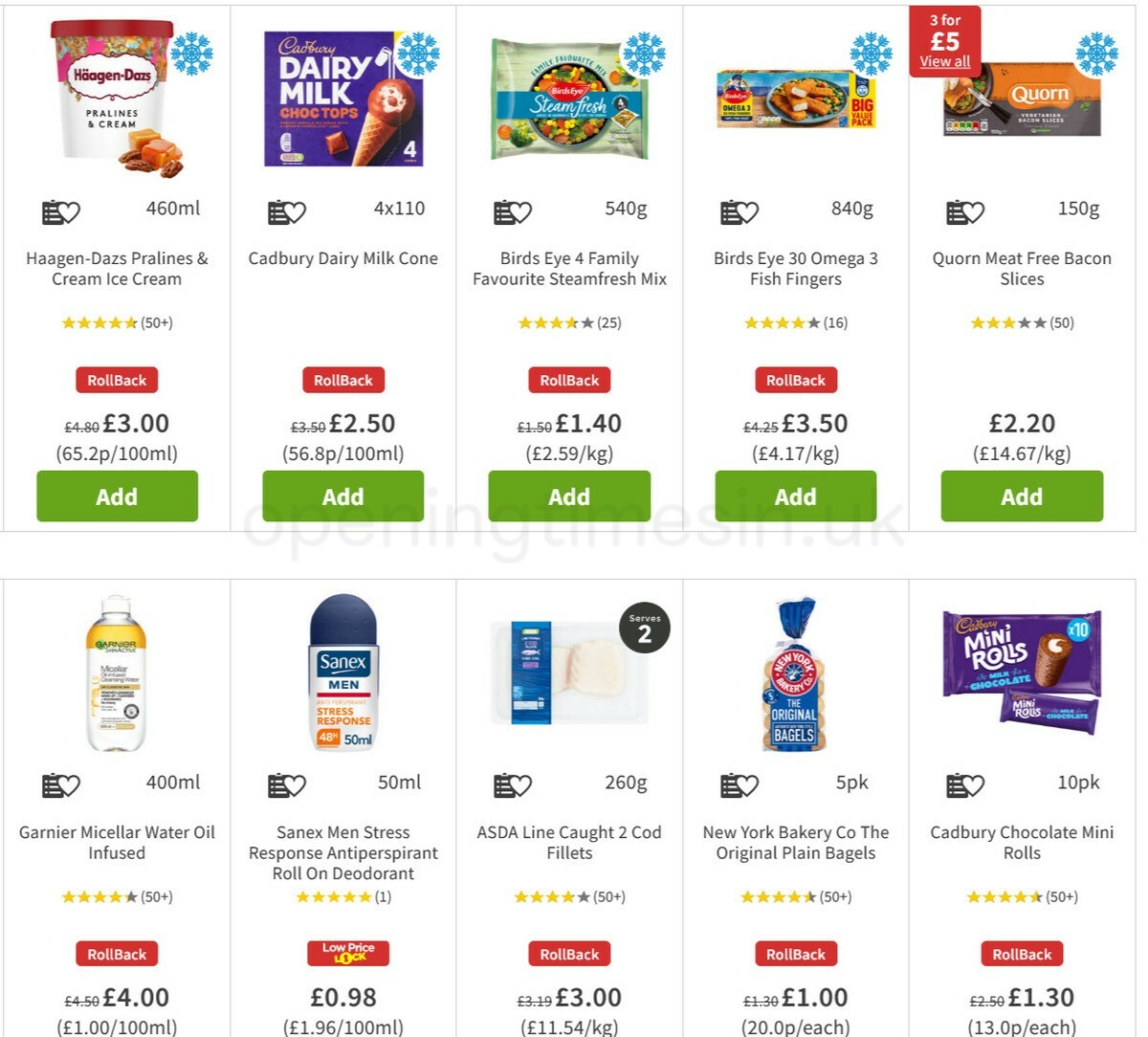This image is a detailed screenshot of a grocery store's online shopping interface, showcasing a variety of products along with their prices, promotional details, and customer reviews. 

**Top Row (Left to Right):**
1. **Haagen-Dazs Pralines and Cream Ice Cream:** 460 milliliters for £3.00, originally £4.80. Price per 100 milliliters is 65.2 pence. Promotion is "rollback". Rating: 4 stars after 50 reviews. An "Add" button is available.
2. **Cadbury Dairy Milk Choc Tonic:** Actually labeled as Choc Tops. Quantity: 4 per box for £2.50. Promotion: rollback.
3. **Bird's Eye Four Family Favorite Steamed Fresh Mix:** 540 grams for £1.40, originally £1.50. A bargain deal.
4. **Bird's Eye 30 Omega-3 Fish Fingers:** £3.50, originally £4.25. Rating: 4 stars from numerous reviews.
5. **Quorn Meat-Free Bacon Slices:** Originally mistaken as having four stars, but actually rated 3 stars. Priced at £2.20.

**Bottom Row (Left to Right):**
1. **Garnier Molecular Water Oil Infused:** On rollback, likely for a reason.
2. **Sanix Men’s Stress Response Antiperspirant Roll-On Deodorant:** Literally one review but a full 5 stars.
3. **ASDA Line-Caught Two Cod Fillets:** £3.00, on rollback.
4. **New York Bakery Company Original Plain Bagels:** Pack of 5 for £1.00.
5. **Cadbury Mini Chocolate Rolls:** Priced at £1.30. All products in this segment are on rollback promotions.

The watermark on the image reads "opening times sin UK".